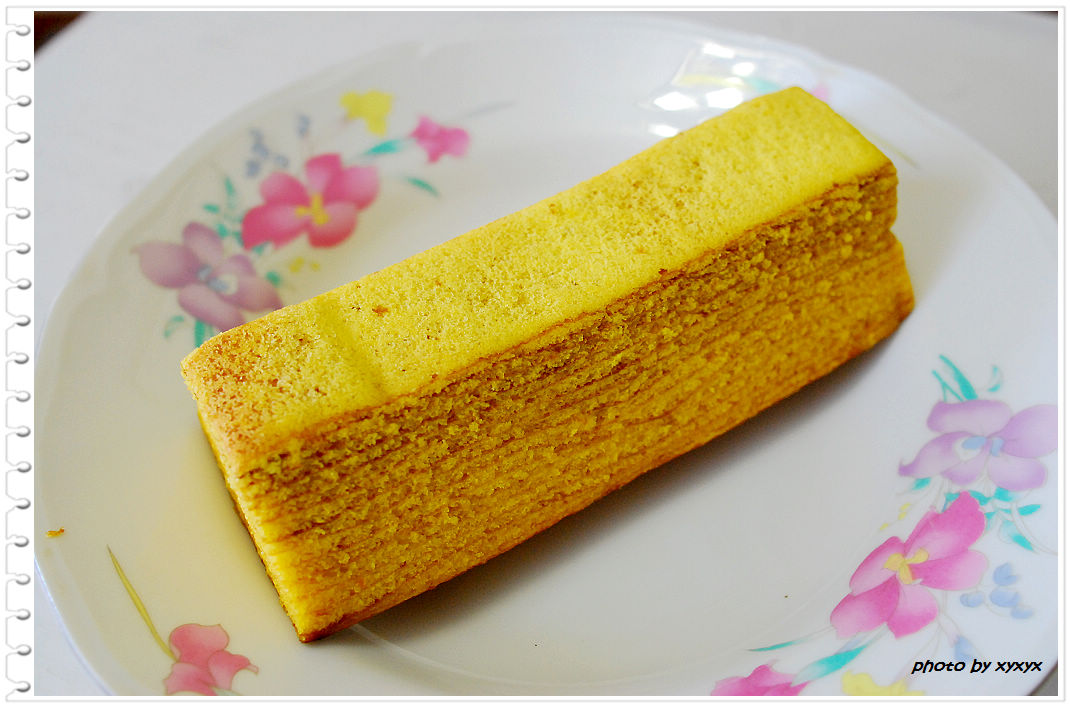The photograph showcases a rectangular, multi-layered, spongy yellow pastry placed on a white plate adorned with various flowers. The floral design includes purple, pink, and yellow blooms accompanied by green leaves and delicate white branches. The plate rests on a white, slightly wrinkled tablecloth that hints at a dark brown table beneath it. In the bottom right corner of the image, "photo by XYXYX" is clearly visible in black text. The photograph's border is outlined with a thin white line.